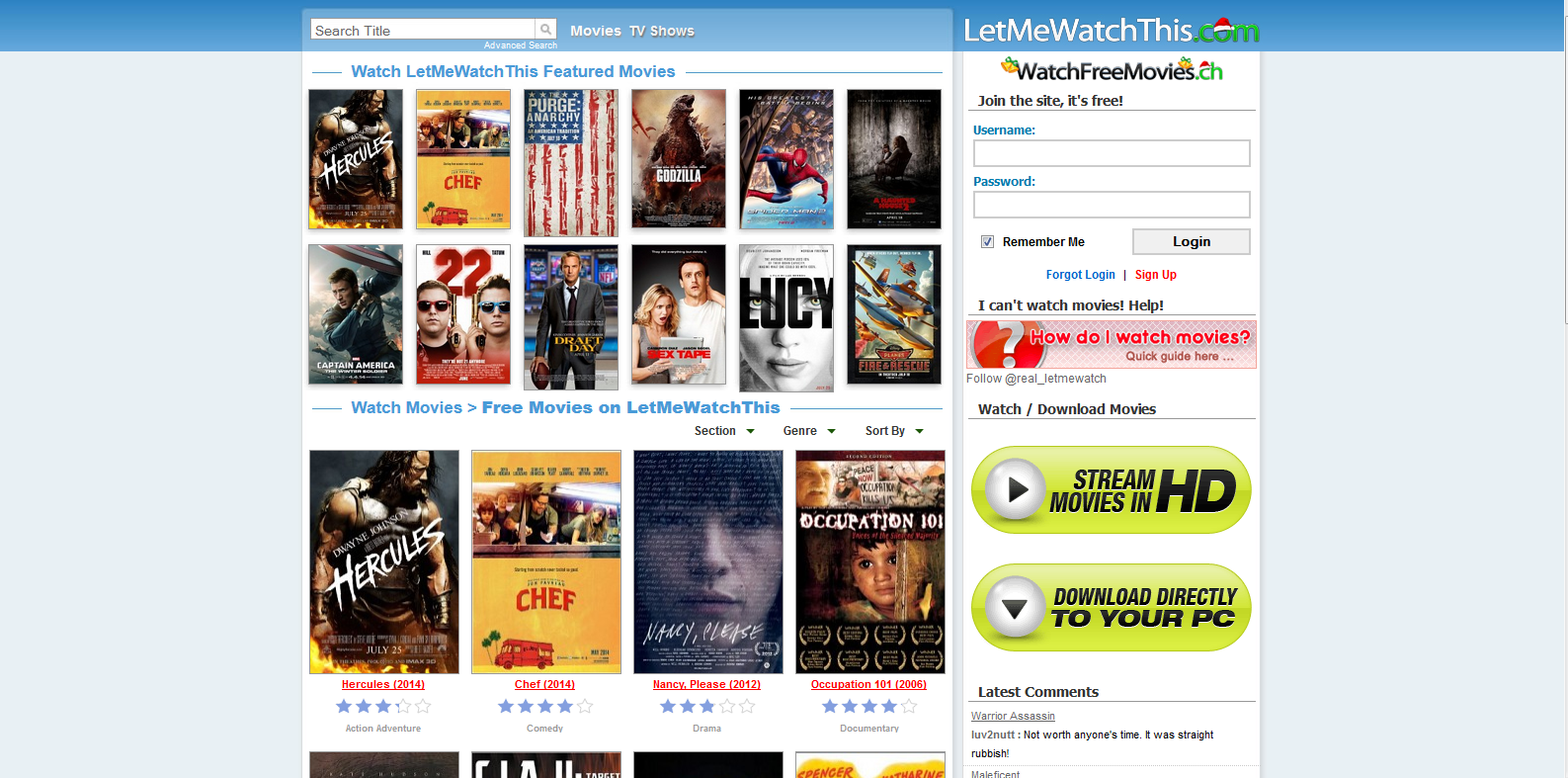The image features a web interface for a movie streaming website. At the top, a blue banner spans across the width of the page. Embedded within this banner, there is a white search box labeled "Search Title" in black text. To the right of the search box, the words "Movies" and "TV Shows" appear in white text. On the far right, the text "LetMeWatchThis.com" is displayed, with the dot "com" in green and the "O" decorated with a Santa hat.

Below the blue banner, the background transitions to white. In blue text, it reads "Watch LetMeWatchThis Feature Movies." Listed below are movie titles such as "Hercules," "Chef," "The Purge: Anarchy," "Godzilla," "Spider-Man," and an unidentified title in red text. 

The row beneath features more movie titles, including "Captain America 2," "Draft Day," "Sex Tape," "Lucy," and "Fire and Rescue." This section also includes a blue instruction text, "Watch Movies, Free Movies," with a reminder, "Don't LetMeWatchThis." The movies listed here include "Hercules," "Chef," "Nancy, Please," and "Operation 101," with their titles highlighted in red.

On the right-hand side of the page, at the top, it reads, "WatchFreeMovies.ch," with "ch" in green letters. Below this, in black text, it states, "Join the site, it's free." Further down, in blue text, there is a "Username" label followed by an entry box. Below that, there is a "Password" label with another entry box for users to input their information.